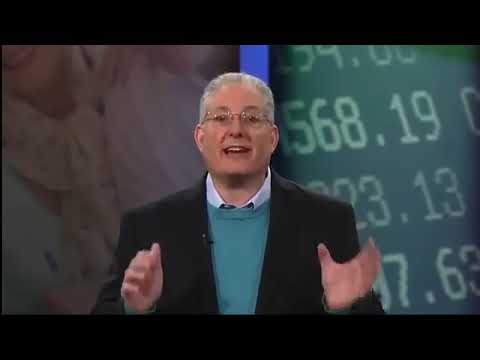A small square image features an older man, likely in his 60s, standing and speaking directly towards the camera. His mouth is open, revealing the top row of his teeth as he speaks. He wears wire-rimmed glasses and has short, slicked-back grayish-white hair. The man is dressed in a black or dark gray suit jacket over a blue sweater vest and a white collared shirt. A small microphone is attached to the lapel of his jacket. His hands are in motion, with his right fist partially closed and his left hand open, facing the viewer. The image is framed by solid black horizontal strip borders at the top and bottom. Behind the man, the background is divided into three sections: a brown marbled pattern on the left, a vertical blue line in the center, and a green field with rows of light green numbers like a stock ticker on the right, with "568.19" among the visible figures. The overall image carries a broadcast-like quality, with a slight blur, particularly around his moving hands.